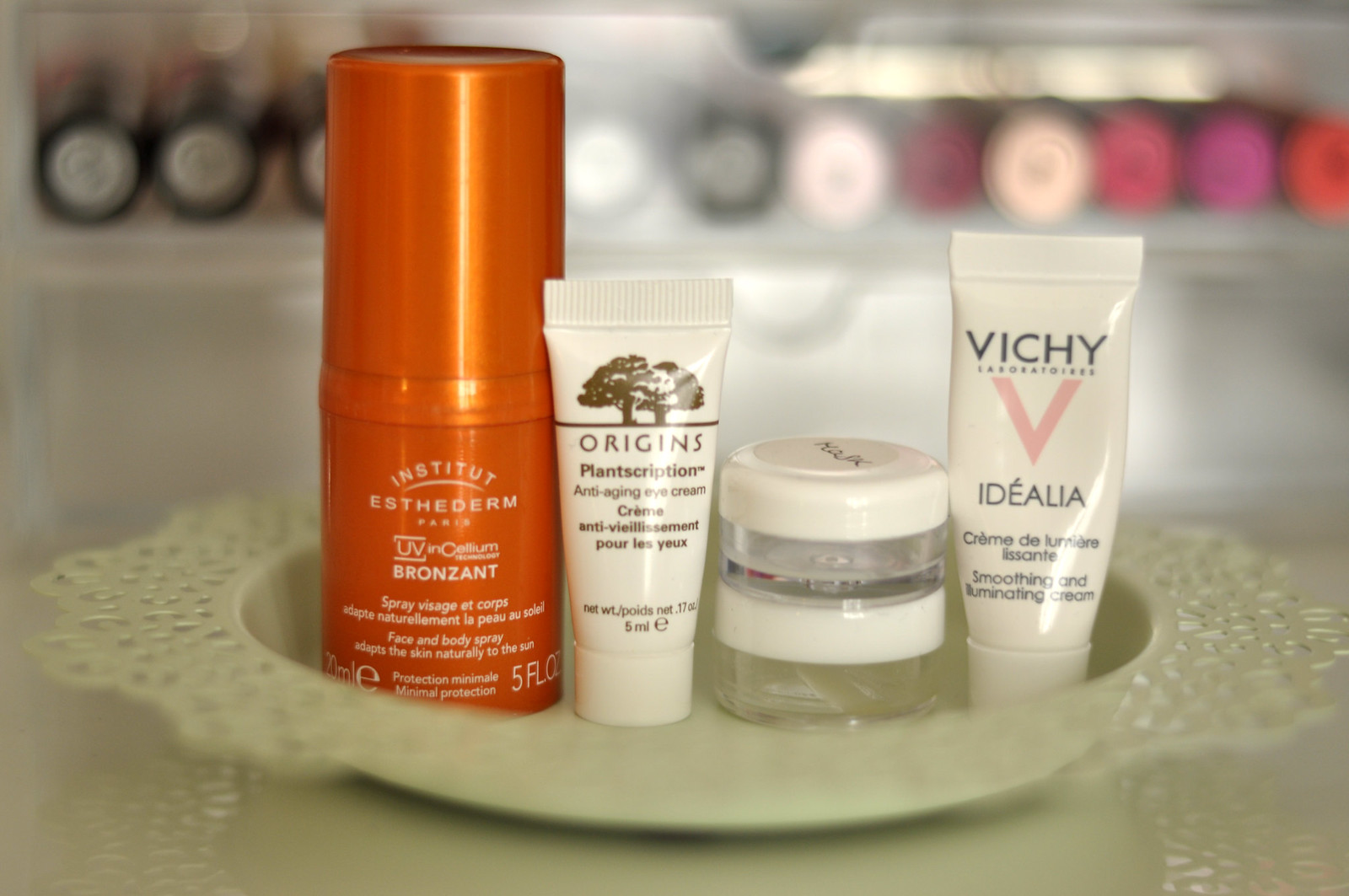In the center of this photo is a modestly sized white bowl containing an array of four distinct items. To the left, there is an orange bottle approximately five inches tall. The bottle is labeled in a unique manner with the text "Institut Esthederm" prominently displayed underlined, accompanied by "UV Bronzant" indicating it is a face and body spray with a capacity of five fluid ounces. Moving inward, we encounter a small white bottle adorned with a brown tree emblem on the front, clearly marked "Origins Plantscription Anti-Aging Eye Cream," also containing five fluid ounces. Adjacent to this is a pair of stacked jars, each filled with a clear liquid and capped with white lids. Finally, to the far right stands another bottle of lotion, similar in size at about five inches tall, labeled "Vichy" in black text with a pink "V" beneath it. The meticulous arrangement and diverse collection of skincare products create an intriguing display within the elegant white bowl.